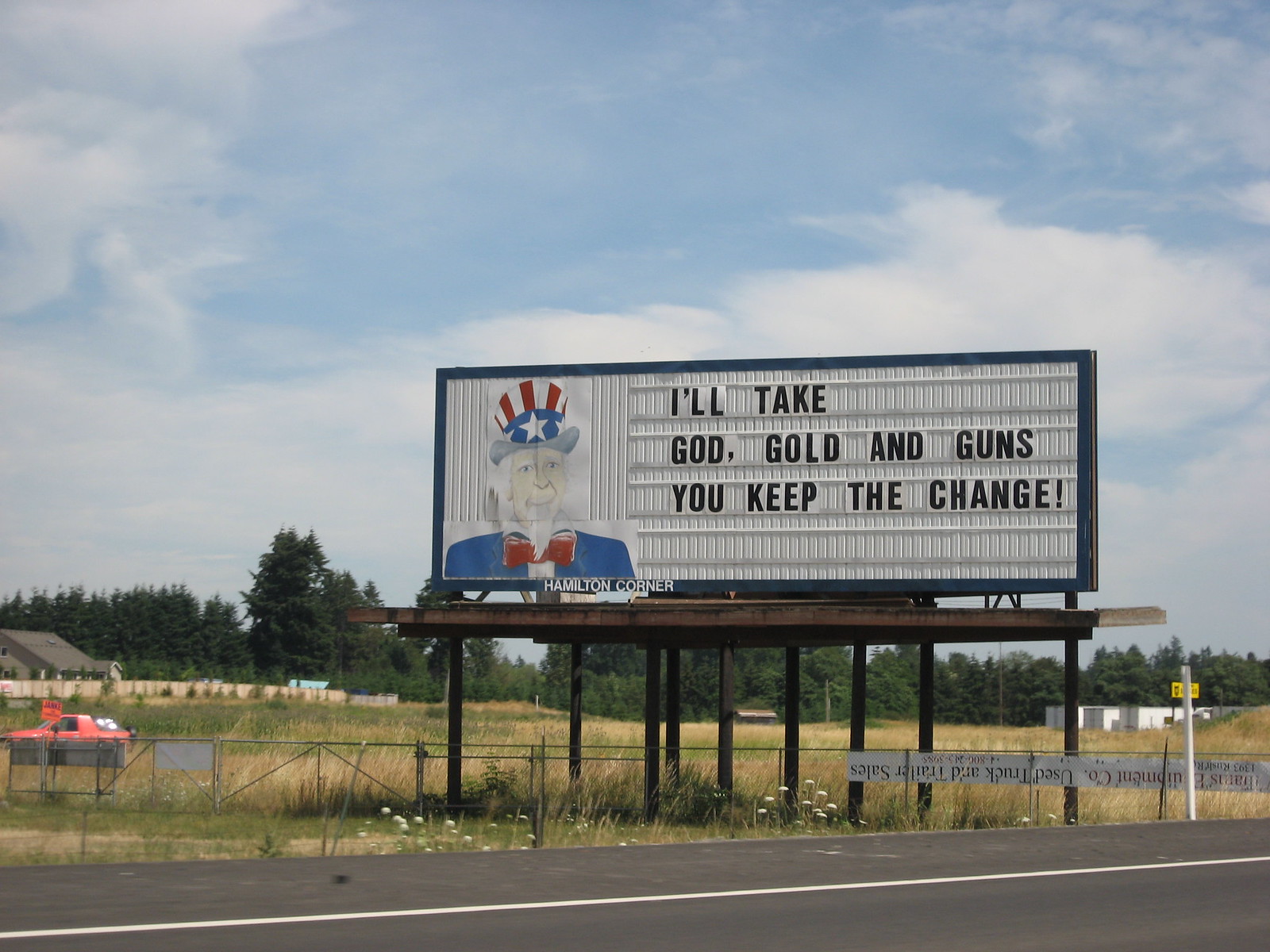A vibrant image portrays a scenic scene along a bustling highway. In the foreground, a small field stretches out, bordered by a weathered fence bearing a modest sign. The sky above is a brilliant blue, adorned with fluffy white clouds that enhance the picturesque setting. A vivid red car is seen driving behind the fence, adding a pop of color to the composition. 

In the background, vast greenery unfolds with a sprawling field leading up to a charming house surrounded by numerous trees. Further back, several large trucks are visible, indicative of the highway's activity. Dominating the scene is a massive roadside sign on sturdy brown wooden legs, making a bold statement. The sign, set against a white background, features an iconic image of Uncle Sam dressed in red, white, and blue. In bold black print beneath the image, the phrase "I'll take God, gold, and guns, you keep the change" is prominently displayed. 

This entire scene, captured from a vantage point beside the highway, exudes a sense of Americana and the varied landscapes of the countryside, making it highly visible to all passersby.